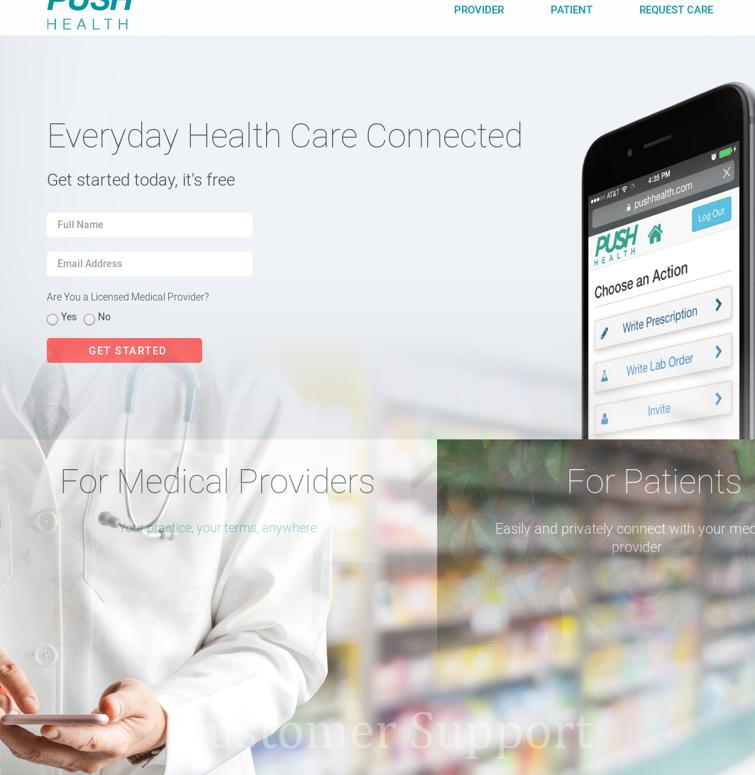This is a detailed screenshot of the main page of the Push Health website. On the right side of the screen, there is an image of a mobile phone displaying the Push Health logo, which consists of the word "PUSH" in turquoise green italics, with each letter capitalized. Below "PUSH," the word "Health" is written in standard font. The mobile phone screen also shows a menu titled "Choose an Action," with options to "Write a Prescription," "Write Lab Order," or "Invite."

The main section of the webpage features bold black text that reads, "Everyday Health Care Connected," followed by an invitation to "Get Started Today" with the notice that it's free. Below this, there are two white input fields where users can enter their full name and email address. Underneath these fields, there is a question: "Are you a licensed medical provider?" with circular buttons to select "Yes" or "No."

At the bottom of this section, there is a prominent red button labeled "Get Started." The website is designed to cater to both medical providers and patients, offering the option to click on either "Provider" or "Patient" to continue.